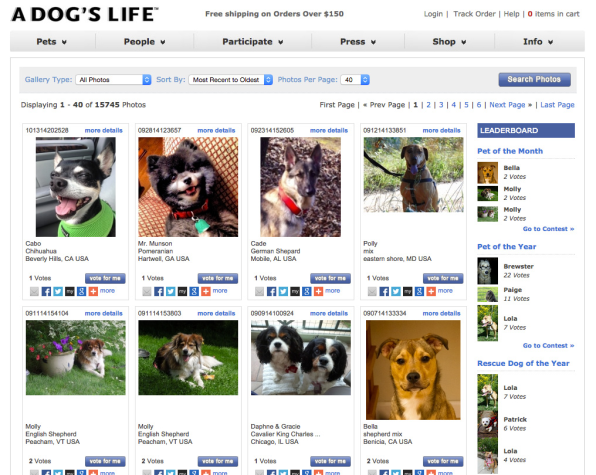The image depicts a website titled "A Dog's Life," with the title prominently displayed in bold, capital letters at the top left of the screen. At the top of the page, a banner announces "Free shipping on orders over $150." Adjacent to this banner are navigational links allowing users to login, track orders, or seek help. A cart icon indicates "0 items in cart."

The webpage features a collection of dog photos, each accompanied by descriptive text and a "Vote for Me" button. Above each photo, there is an option for "More details," a unique identifying number, and the state where the dog is located. This suggests the site is not for purchasing dogs, but rather a platform for voting in some form of competition.

On the right side of the webpage, there are leaderboards showcasing categories such as "Pet of the Month," "Pet of the Year," and "Rescue Dog of the Year," further implying a voting or ranking system rather than an e-commerce site.